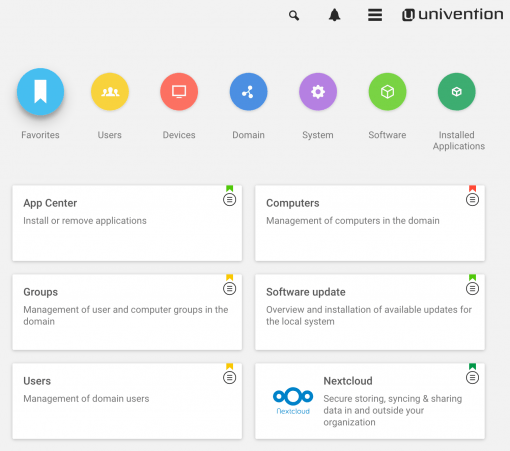The image appears to showcase a digital interface, likely for a software application or system management tool, referred to as "uni-vention." The interface features an "App Center" and several color-coded buttons that organize different functions. There is a purple button labelled "Installed Applications," a blue button for "Domain," and a yellow button that seems to be for "Users." The layout displays a variety of colors and categories, each button representing a specific system function or group, and suggests a user-friendly, visually organized method for navigating and managing the system's features.